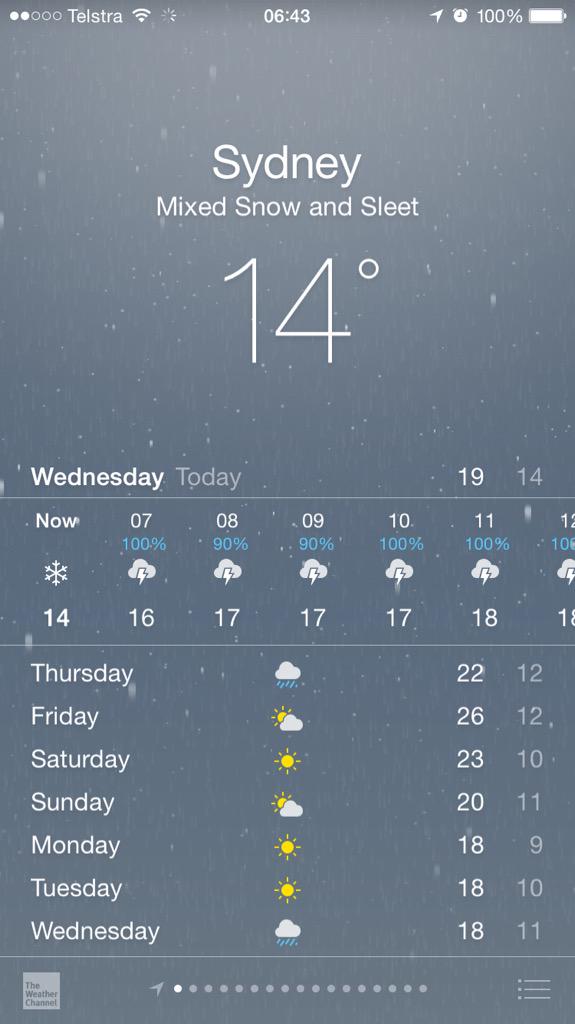The image displayed on a mobile phone shows a detailed screen capture of a weather app for the city of Sydney. At the top of the image, the time is indicated as 6:43 AM, the battery is fully charged at 100%, and the service provider is Telstra. Additionally, there is a Wi-Fi connection signal displayed.

The weather app reports that Sydney is currently experiencing a mix of snow and sleet, with a temperature of 14 degrees Celsius. The background of the app indicates rainfall, suggesting that it is raining at the moment. The date is highlighted as Wednesday, the 6th of the month.

The weather forecast for the upcoming days is as follows:
- Thursday: Rainy
- Friday: Cloudy
- Saturday: Sunny
- Sunday: Cloudy
- Monday: Sunny
- Tuesday: Sunny
- Wednesday: Rainy again